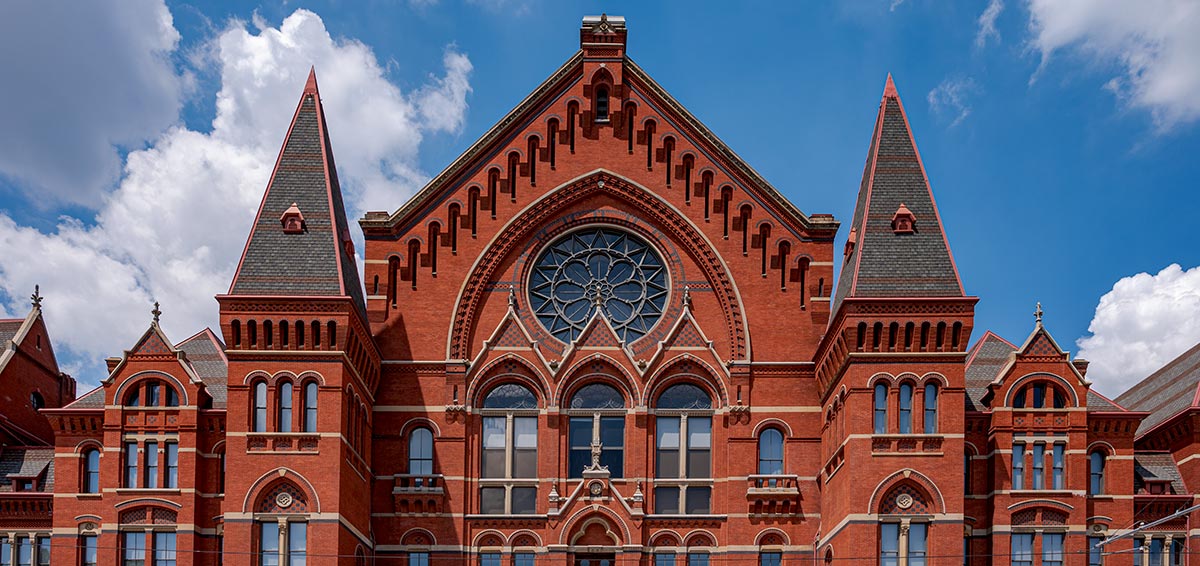This is a color photograph taken on a bright, sunny day, featuring the top portion of an aged, redbrick building with intricate architectural details. The image is in landscape mode, emphasizing the building's elaborate structure against a background of a blue sky dotted with fluffy white clouds. The central focal point is a large, round window adorned with ornate, flowery designs. Flanking the window are several tall, skinny windows with rounded arches. The building also features multiple sharp, pointed towers and steeple-like structures with dark tops, lending to its grand and impressive appearance. Despite resembling a church, the absence of crosses suggests it could be part of a university or another historical complex. The windows, with their navy-blue and blackish hues, together with the vibrant blue sky and the interplay of shadows on the left, enhance the building's majestic presence.